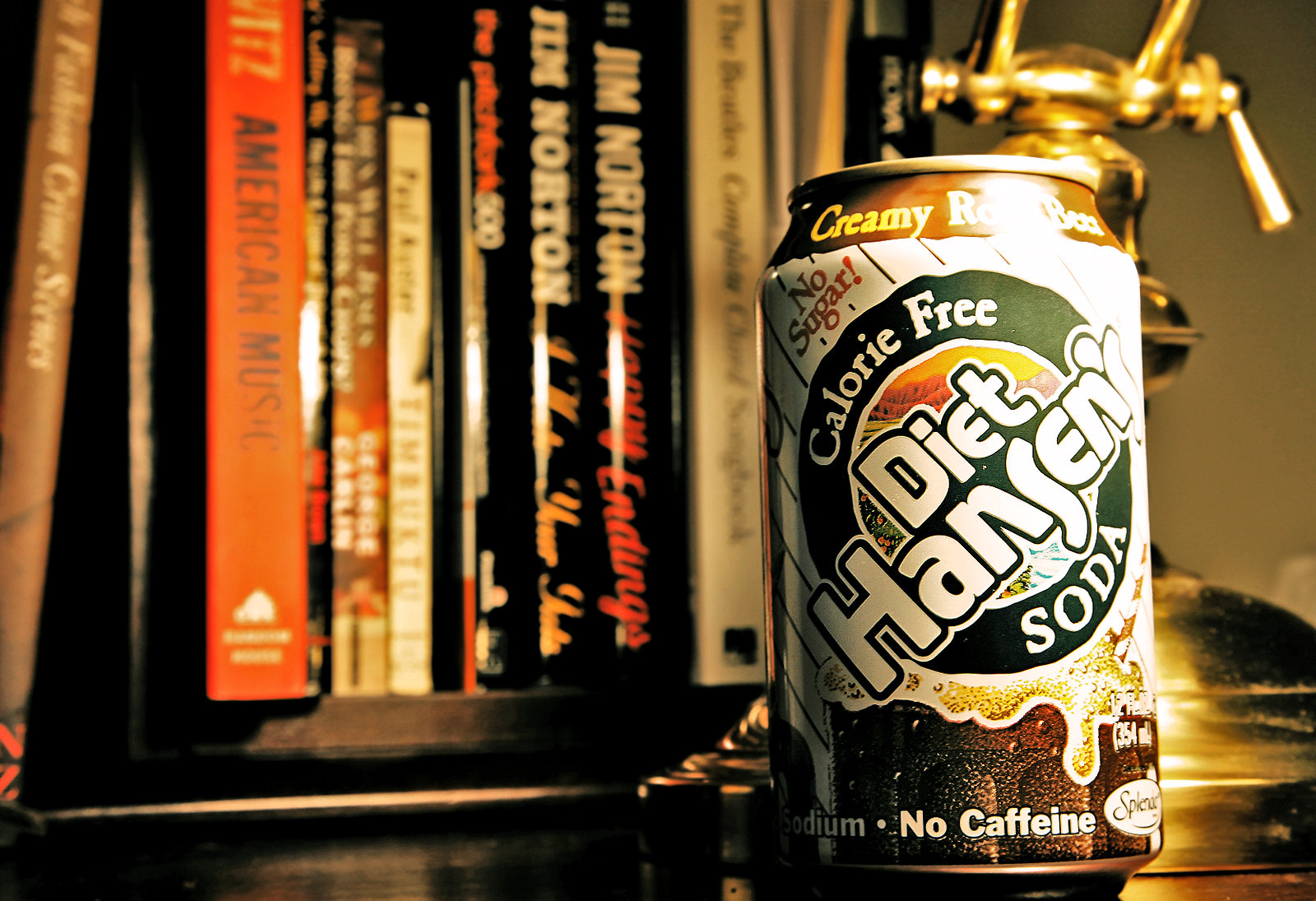This detailed color photograph prominently features a can of Diet Hansen's creamy root beer soda placed on what appears to be a table in front of a fully stocked bookshelf. The can itself is designed with a combination of white, green, yellow, and brown colors. It has a light brown strip around the top, where the words "creamy root beer" are written. Below the brand name "Diet Hansen's," which is printed diagonally in white letters outlined with green, there's an olive green circle containing the text "calorie free" and "soda." At the bottom, the can is labeled “no caffeine.” The backdrop of the image includes a bookshelf filled with books of various colors, including brown, orange, white, and black covers with different text and authors visible. Notably, one book spine displays the title "American Music," and a couple of books are authored by Jim Norton. The photograph’s primary focus is the single can of root beer soda, contrasting against the array of books behind it.